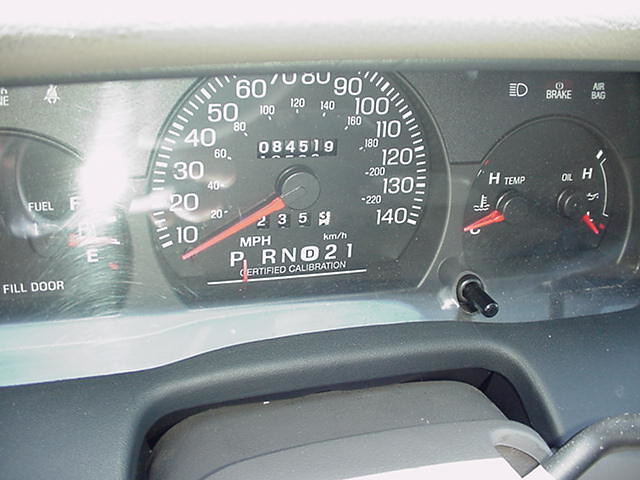The image depicts the dashboard of a car, showcasing a comprehensive view of the speedometer and other essential gauges. To the left of the speedometer, the fuel gauge is visible, indicating the car's current fuel level. Adjacent to the speedometer, various other instrument readings are displayed, including the car's mileage, which reads 84,519 miles. Below the mileage, the gear indicator is visible, showing the current gear of the vehicle. Additionally, there are some numbers visible on the dashboard that seem to read "2, 3, 5, 3," but their exact purpose or context is not clearly specified.